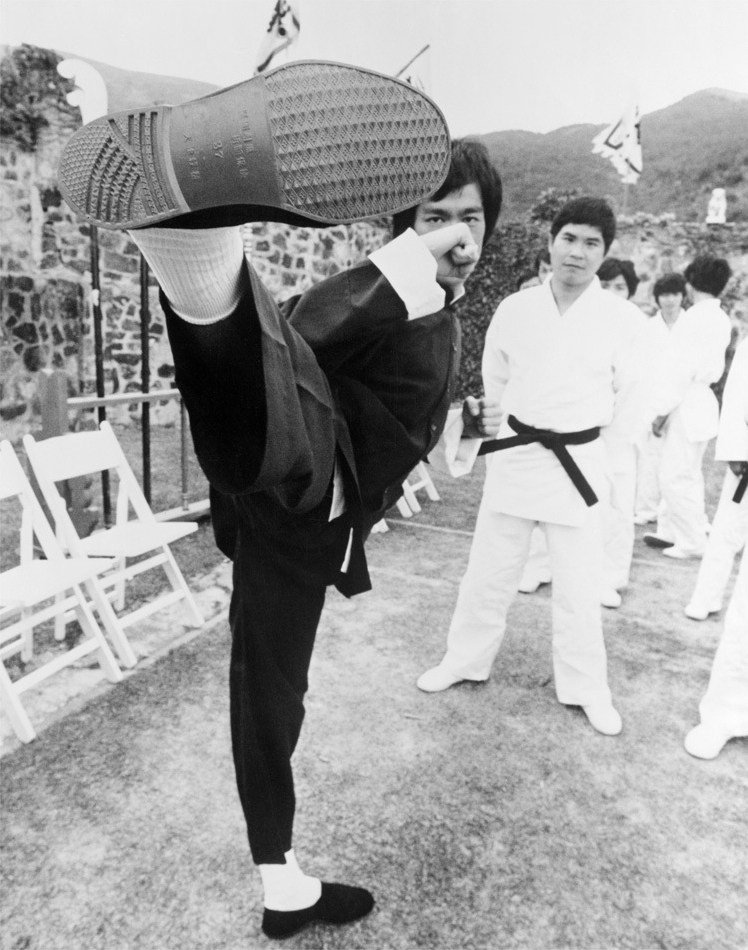This black and white photograph, seemingly taken in an outdoor training area or dojo set against a backdrop of rolling hills and sparse trees, prominently features Bruce Lee in the center-left. Bruce Lee, dressed in a traditional black kung fu suit with white cuffs and a front button closure, is captured in mid-motion performing a high vertical kick towards the camera. His right foot extends upward, revealing a black rubber sole, while his left foot maintains balance on the ground. His right hand, clenched in a fist, partially obscures his face, and his other hand rests near his waist. 

Surrounding Bruce Lee, a group of men in white martial arts uniforms with black belts stand attentively, their white shoes and focused gazes pointing towards him. The scene also includes various elements such as a brick wall to the right, a few foldable chairs on the left, and a series of flags on tall poles behind the martial artists, though the wind has wrapped them, making their designs obscure. In the distance, the landscape features a mountainous area under a clear sky, enhancing the serene yet intense atmosphere of this dynamic outdoor setting.